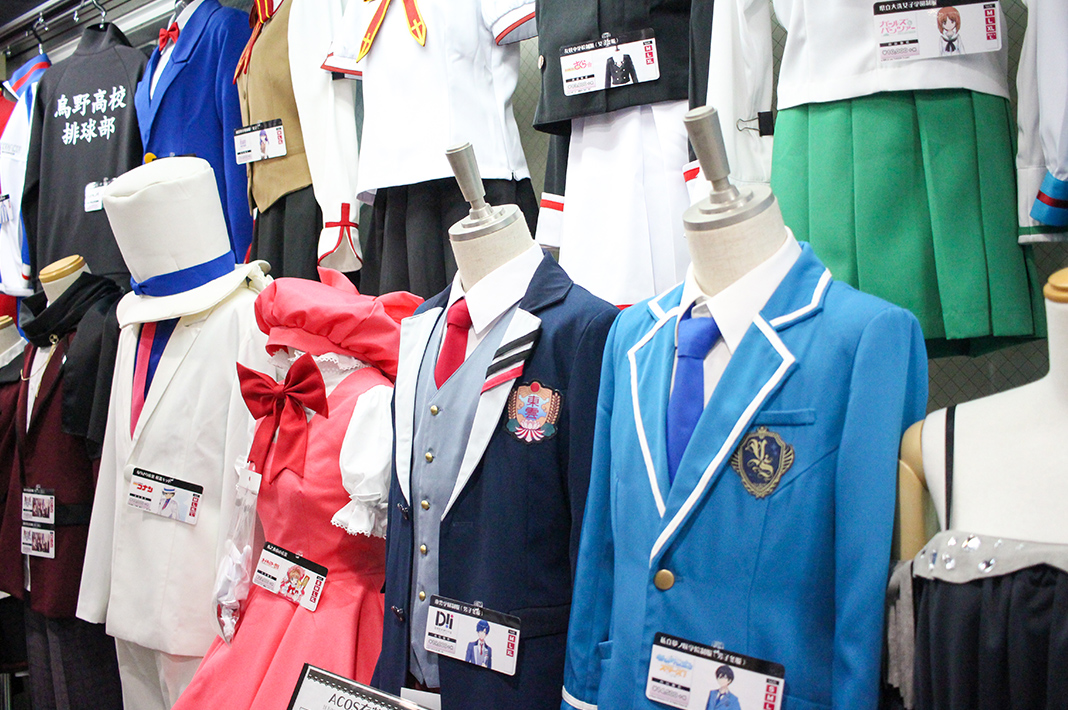The photograph captures a meticulously arranged display of cosplay costumes, most of which are school uniforms inspired by various anime characters. The display features multiple headless mannequins positioned in two rows, each adorned with costumes that range in color and style from blue and dark blue blazers to pink and green skirts. Each costume is accompanied by a card with text—likely in Japanese—corresponding to the character it represents. Notable outfits include a distinctive red vest with a white shirt and black cloak, as well as a white business suit with a pink tie, complemented by a large white tall hat with a blue band and a blue shirt. The mannequins, crafted from silver dowels protruding from their necks, create an intriguing and cinematic visual impact. The carefully labeled attire, complete with detailed descriptions, suggests that this display could be situated in a shop, museum, or studio, shedding light on the intricate art of anime cosplay.